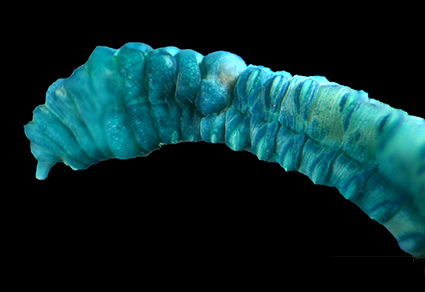The image displays a close-up photograph, likely taken under a microscope, portraying a blue-green segmented object that curves from the lower right-hand side to the left middle of the frame. The object resembles an appendage of an insect or possibly a sea creature, characterized by its narrow, elongated shape and segmented structure with darker lines between the segments. The overall coloration includes hues of light blue, teal, and pale green, giving it an almost iridescent appearance. The background is stark black, creating a striking contrast that emphasizes the intricate details and curvature of the object. Some segments appear to be larger and more curved than others, while some are flatter. The image has a surreal and somewhat mysterious quality, evoking the style of a meticulously crafted painting.